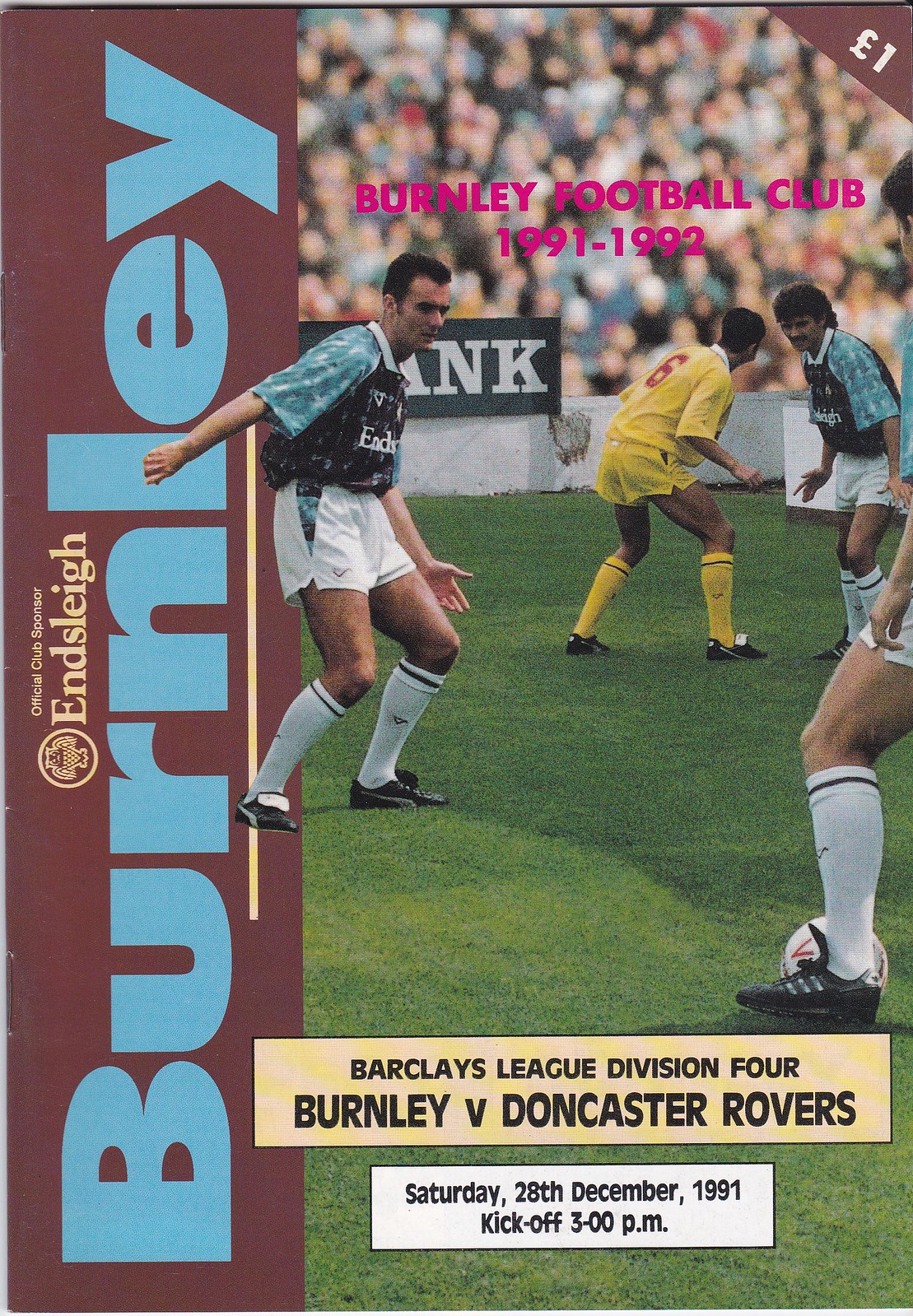The image depicts a cover for a football program from Burnley Football Club for the 1991-1992 season. The left side features a vertical purple strip with the name of the magazine, "Burnley," written vertically in blue. Above this, "Endersley" is written in yellow. Further down, the text reads "Official Club Sponsor," followed by "Sly, Burnley." On the right side of the cover, a photograph shows football players on the field. One team wears a black and light blue shirt, white shorts, white socks, and black shoes, while the opposing team is clad in all yellow. At the top of the cover, in pink text, it states "Burnley Football Club 1991-1992." At the bottom, it reads "Barclays League Division 4, Burnley versus Doncaster Rovers, Saturday 28th December 1991, kick-off 3.00 pm." In the top right corner, the price is marked as "Euro 1."